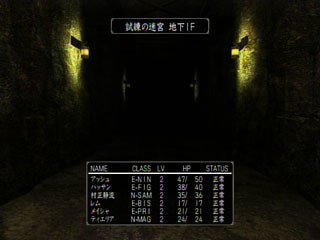This image is a small, dimly lit screen capture from a computer game, with most of the screen enveloped in darkness. We appear to be gazing down a narrow, shadowy hallway that is barely visible. Illuminating the scene, two wall sconce lamps on either side emit a soft yellow glow, casting circular patches of light on the walls. At the top of the screen, a box displays text in Asian characters, providing information relevant to the game. The bottom of the screen features a larger information panel, organized with headers such as "Name," "Class," "Level," "HP," and "Status." This panel contains a mix of Asian characters and English letters, with numerical values listed under the "HP" column, offering detailed stats about the character being depicted.